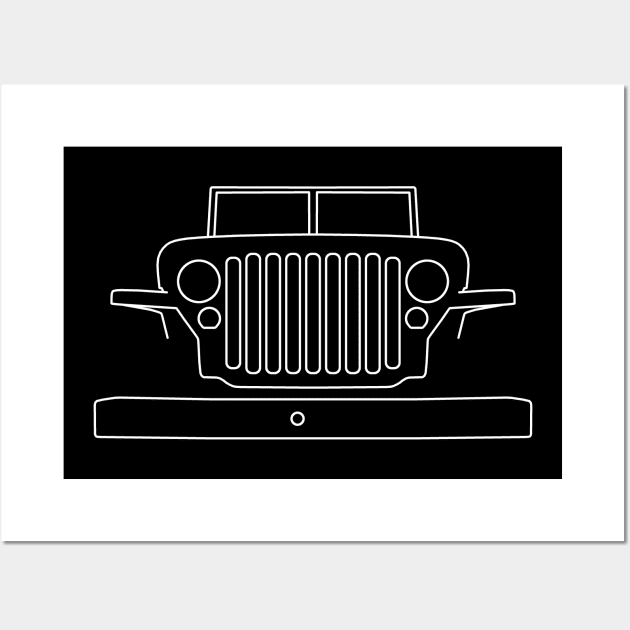The artwork is a minimalist black and white lithograph of a vintage car's front grill. The piece is rendered on a black background and features a thin white line drawing of the car's frontal view. The car illustration shows a distinctive split windshield, a prominent grill, two large headlights, and two smaller lights positioned below the main headlights. Extending horizontally at the bottom is a rectangular bumper with a small circle at its center, which may suggest a classic car logo or emblem. The grill area is accentuated by what appear to be protruding "ears," possibly representing wheel covers. The entire composition is bordered by a thick white frame and is showcased against a white wall, emphasizing its clean and simple aesthetic.